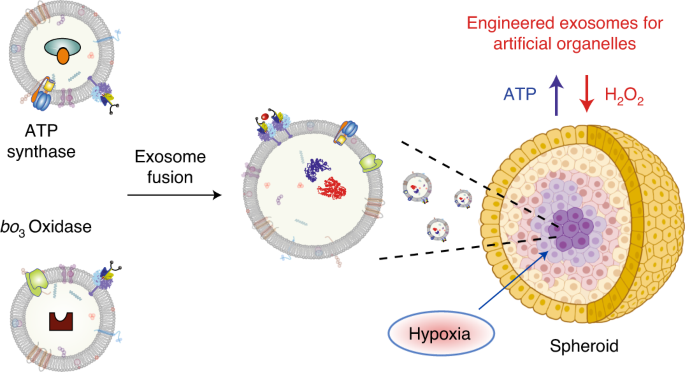This detailed scientific diagram illustrates various phases of the transformation of an organic compound within cellular biology. At the left side, the process begins with ATP synthase and BO3 oxidase. As these enzymes undergo exosome fusion, they lead to the formation of a hypoxia-related spheroid structure. The spheroid appears yellow with a honeycomb outer layer and a purple interior, indicative of its complex internal composition. The caption “engineered exomes for artificial organelles” is prominently featured at the top. This biological reaction highlights the increase of ATP and the decrease of H2O2 within the system. The intermediate structures, depicted in shades of gray with blue and green organelles, further emphasize the stages of ATP synthase and oxidase in the conversion process. This high school or community college-level illustration showcases the intricate process of creating larger cellular spheroids through exosome fusion for the application of artificial organelle engineering.